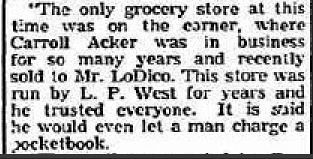The image is a small, rectangular section that appears to be clipped from a newspaper. It features a white background with a thin black line outlining the left, bottom, and right edges, leaving the top open. The text, which is slightly blurry and in black font, reads: "The only grocery store at this time was on the Erna, where Carol Acker was in business for so many years and recently sold to Mr. Lodico, L-O-D-I-C-O. This store was run by L.P. West for years, and he trusted everyone. It is said he would even let a man charge a pocketbook." The words are enclosed in quotation marks.